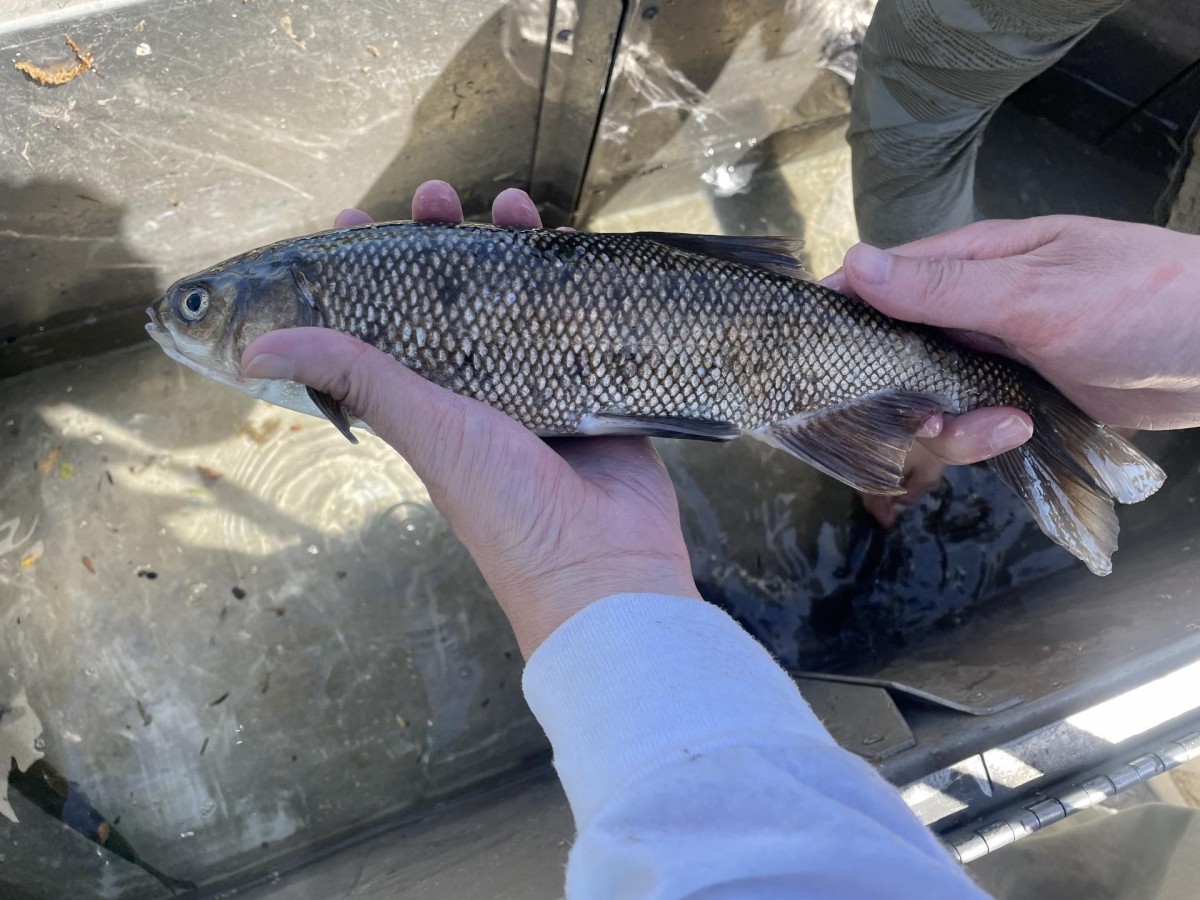The full-color photograph, taken outdoors during the daytime, features a Caucasian male holding a fish inside what appears to be a boat. The man, dressed in a light blue long-sleeve shirt, is holding a slender fish with brown and gold scales. In his left hand, he supports the fish just behind its head, while his right hand grasps its tail. The fish is approximately one foot long and likely weighs only a few pounds. Reflections of water are visible, indicating a body of water nearby, and some water has pooled at the bottom of the boat. Additionally, the upper right-hand corner of the photograph shows part of another person’s leg, suggesting someone else is present but partially out of frame.